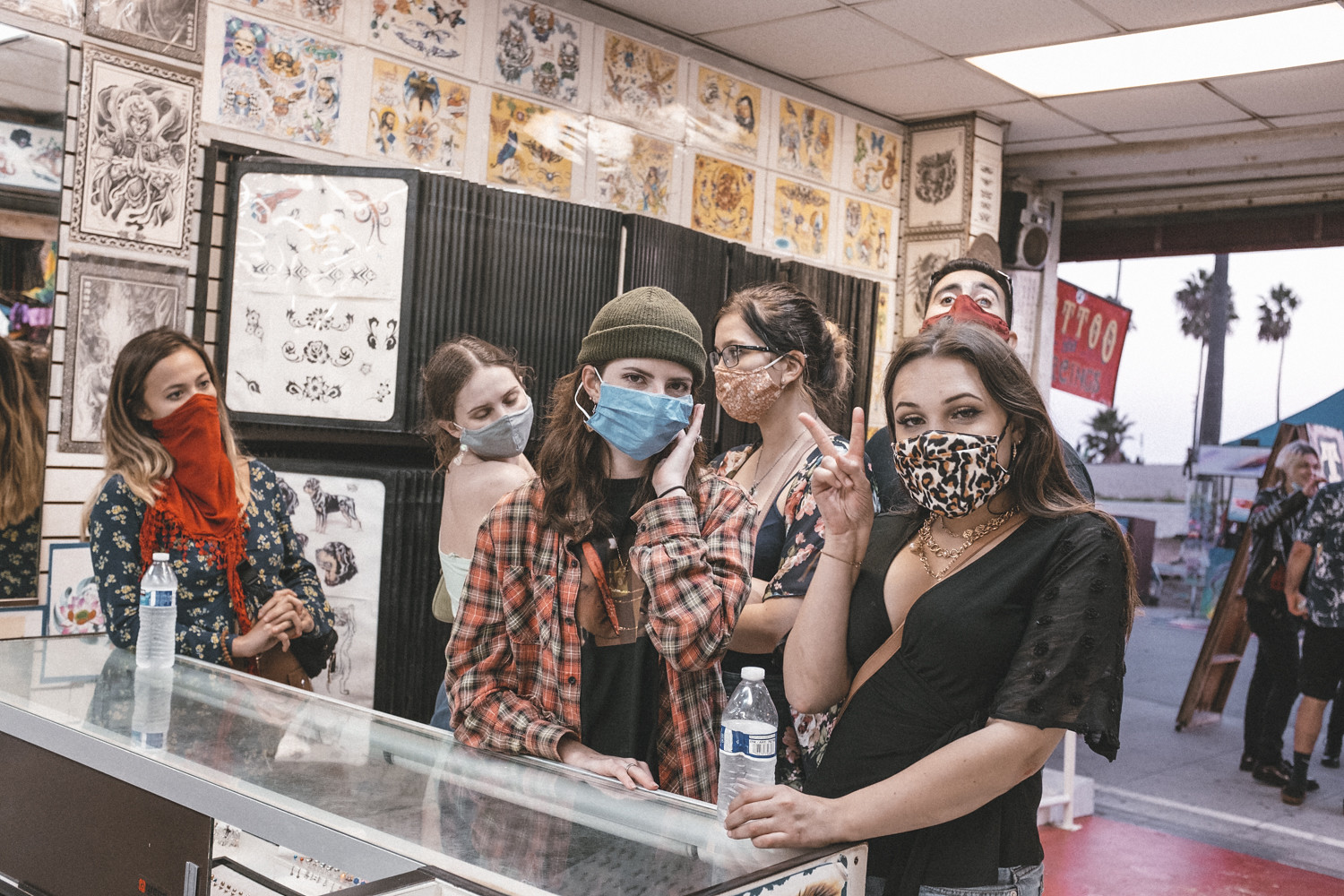The image depicts a group of five women inside a bustling, brightly decorated tattoo shop, likely during the COVID-19 pandemic as they are all wearing various masks. The shop's interior features a vibrant red floor and an open back wall revealing a glimpse of another group of people outside, along with visible greenery and palm trees. Prominently featured is a glass display case filled with tattoo designs, and wall panels also showcasing numerous tattoo flashes. Each woman is uniquely dressed: one in a leopard print mask, black shirt, and making a peace sign while adorned with gold earrings and a chain necklace; another in a plaid shirt, green beanie, and a blue mask with her hand raised to her face; a third in a floral shirt with a pink mask; another in a white halter top with a gray mask; and the last in a red mask and floral top. The vivid ambiance is heightened by flashes with yellow and white backgrounds and the colorful attire of the women, adding to the lively atmosphere of the tattoo shop.